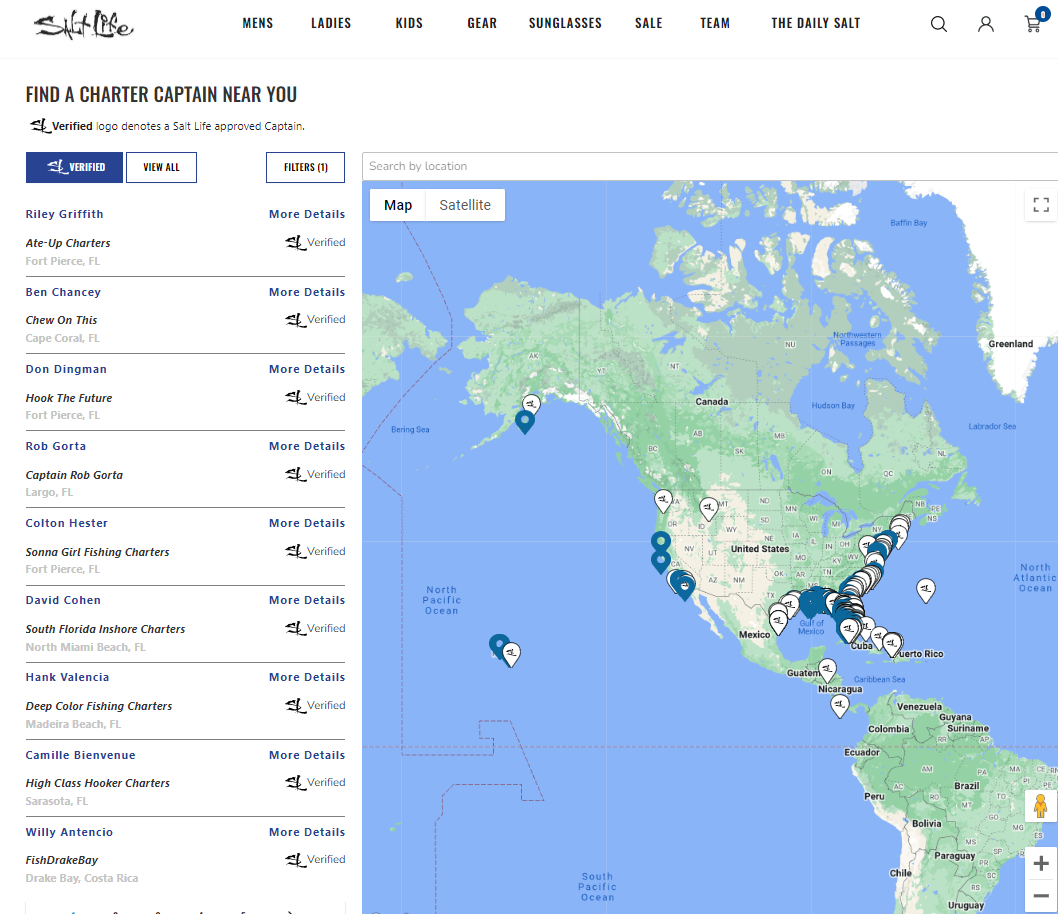The image is a screen capture of a web page from the "Salt Life" website. In the upper left corner, the "Salt Life" logo is prominently displayed in a stylized, fanciful font. Running horizontally across the top of the page are various navigation links for different sections of the website, including "Men," "Ladies," "Kids," "Gear," "Sunglasses," "Sale," "Team," "The Daily," and "Salt." 

On the left side of the image, there is a section with the text "Find a charter captain near you" written in black on a white background. This message is accompanied by a disclaimer, noting that a verified logo identifies a Salt Life-approved captain. Below this text, there is a list of several charter captains' names.

To the right side of the image, a detailed map of North and South America is displayed. The map features a green landmass surrounded by the blue waters of the Atlantic and Pacific oceans, providing a geographic context for the listed charter captains.